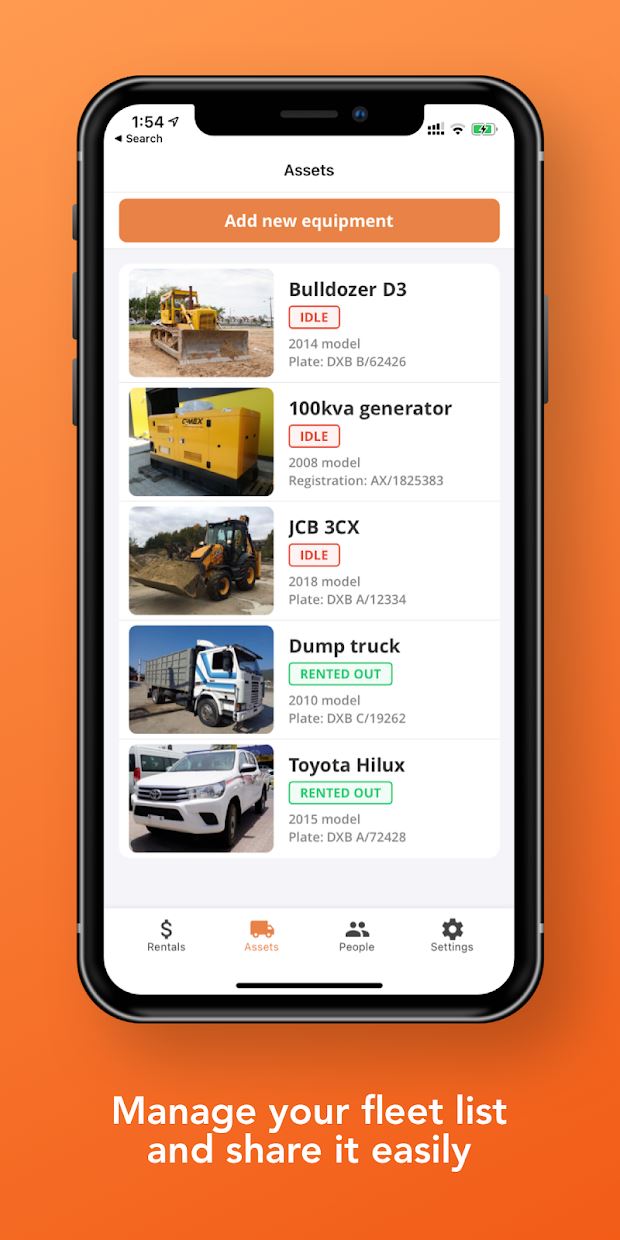This image appears to be an advertisement for a fleet management app. It is designed as a tall, upright rectangular box with an orange background. The focal point is a smartphone displaying the app’s interface. 

On the phone screen, there is a heading labeled "Add New Equipment" with a clickable button. Below this, various pieces of equipment are listed, including a bulldozer, a generator, a dump truck, and a car. Each item shows its current status, indicating whether it is idle or rented out. Equipment that is currently rented out features a green "Rented Out" button next to its picture.

At the bottom of the phone screen, there is a navigation bar with icons labeled "Rentals" (accompanied by a dollar bill sign), "Assets" (with a little truck icon), "People," and "Settings." Notably, the truck icon is orange, suggesting that "Assets" is the active screen in the app.

The bottom of the advertisement features the slogan, "Manage your fleet list and share it easily," emphasizing the app's utility for fleet management. This image effectively showcases the app's features and ease of use, targeting potential users who need to manage and monitor equipment rentals efficiently.